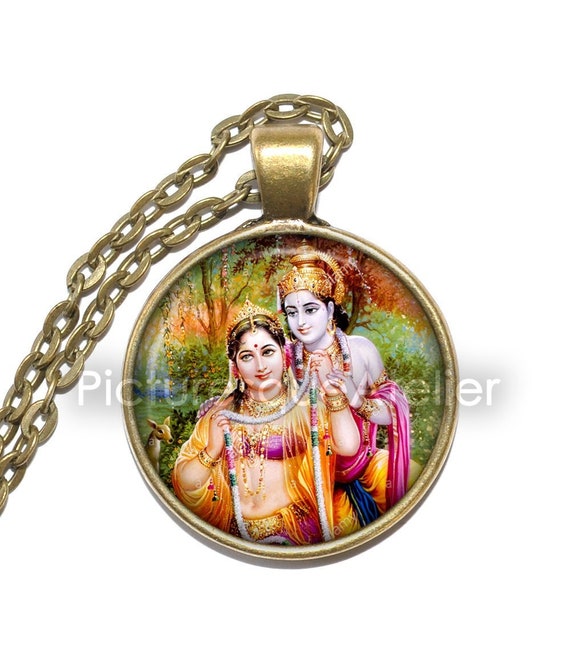This detailed and ornate image depicts a piece of old-fashioned jewelry featuring a large, golden medallion at its center, suspended from a substantial golden chain. The medallion, likely Indian in origin, displays an intricate drawing of two ornately dressed women. Both women are adorned with significant jewelry and wear traditional Indian attire. The woman on the left is holding up a string of beads, predominantly white with green and pink accents, while the woman on the right, draped in a pink robe or cloth over her left arm, touches the other woman's left wrist. She also wears a golden, ornate cap, contrasting with the smaller golden crown on the first woman's head. Both women have a distinctive red dot on their foreheads. The background within the medallion features a serene scene of trees, grass, and a deer on the left side. The piece is framed within a light golden border, and there is an inscription superimposed on the image that reads "PICTURE EQ E AREIELIER" in white text. The color palette includes pink, orange, yellow, white, black, and green. This appears to be a decorative artifact, possibly from a museum or a collection of decorative jewelry.